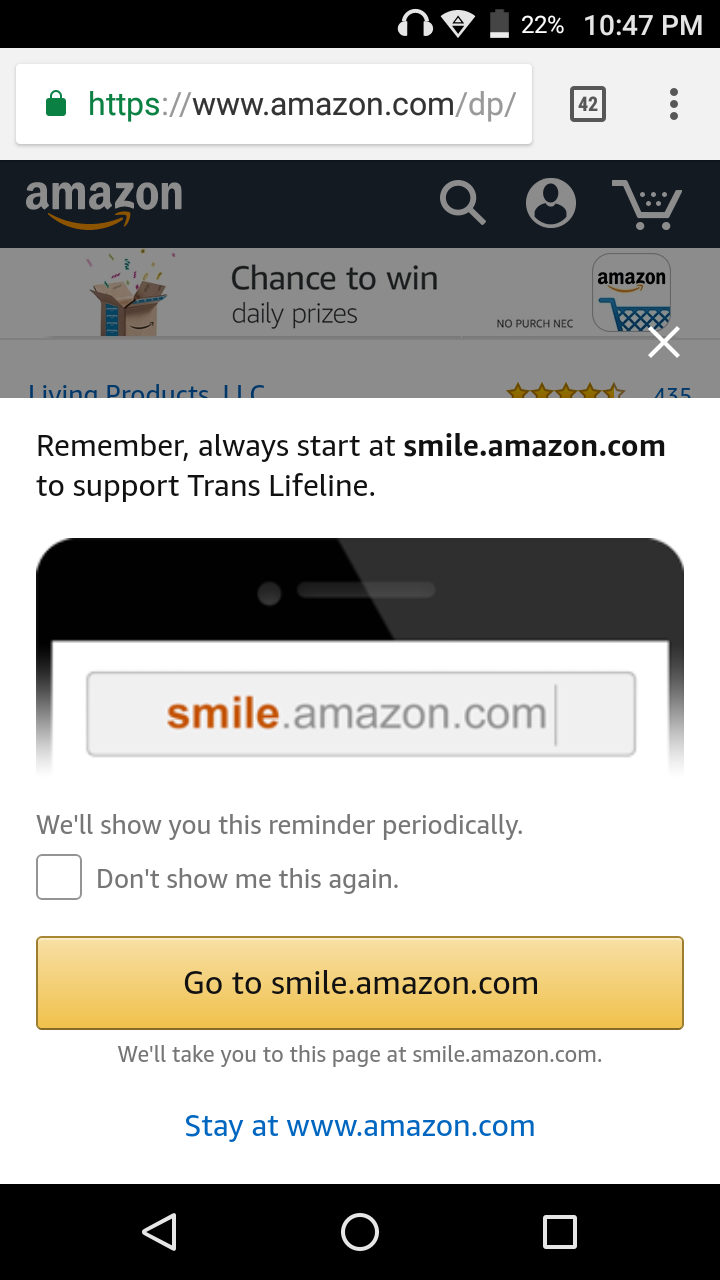This screenshot captures a mobile view of the Amazon website, specifically the support page for Smile.Amazon.com, which encourages users to start their shopping at Smile.Amazon.com to support Trans Lifeline. The reminder box prominently appears with the message: "Remember, always start at Smile.Amazon.com to support Trans Lifeline." Below this message, there’s an unchecked option stating, "Don't show me this again," and a prominent yellow button labeled "Go to Smile.Amazon.com" which redirects the user to the Smile platform. Additionally, there are options to remain on the standard Amazon site with "Stay at www.amazon.com." 

At the bottom left corner, a back button is visible, flanked by a "Go" button in the center and a stop button on the right. The background reveals the Amazon homepage, identifiable by the classic Amazon logo with its distinct orange arrow, a search bar, profile icon, and a shopping cart icon. Details at the top of the screenshot show the time (10:47 PM), the device's battery level at 22%, and that the user is connected to headphones.